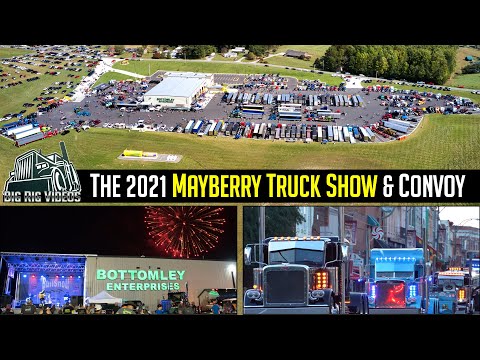The image depicts a detailed flyer for the 2021 Mayberry Truck Show and Convoy. It features a collage of images with black horizontal borders at the top and bottom. In the center, there's a black band with the event title "2021 Mayberry Truck Show and Convoy"; "2021" and "Convoy" are in white text, while "Mayberry Truck Show" stands out in yellow. To the left of the title, there's an illustration of a truck. 

The top half of the image shows an aerial view of a large parking lot filled with semi-trucks and cars, surrounded by a green field with some buildings. A central white building with a flat roof is prominently situated in the parking lot.

The bottom half of the flyer features two distinct photos. The left picture captures a nighttime scene with a black sky lit up by red fireworks. It includes a building with a sign reading "Bottomley Enterprises" and a performance stage to its left, surrounded by lights and tents with people gathered in front. The right photo shows a parade of semi-trucks lined up on a road, set against a backdrop of more trucks and buildings, conveying a sense of celebration and community.